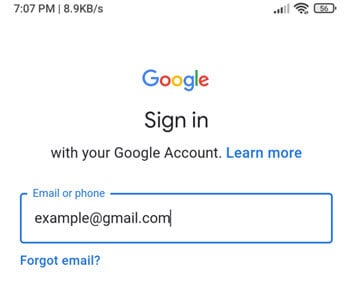The image depicts a cell phone screen with a white background. In the top left corner of the screen, the time is displayed as 7:07 p.m., followed by a vertical bar that shows a data transfer rate of 8.9 kilobytes per second. To the far right, there are icons indicating three out of five signal bars, a full-strength Wi-Fi signal, and a battery level at 56%.

Beneath these icons, the familiar Google logo appears, with each letter in the company's signature colors: a capital blue "G," a small red "o," a small yellow "o," a small blue "g," a lowercase green "l," and a lowercase red "e." 

Under the Google logo, there is an instruction in black text that reads "Sign in." Directly below, in smaller black font, it says "with your Google Account," followed by the phrase "Learn more" in blue letters.

Further down the screen, there is a blue-outlined rectangular input field for an email or phone number. The outline of this field is broken at the top left corner, where it says "Email or phone" in a small font. Within this entry box, the placeholder text "example@gmail.com" is typed in black lowercase letters, with a blinking cursor indicating where additional text can be entered.

Below the input field, in blue text, there is a hyperlink that reads "Forgot email?"